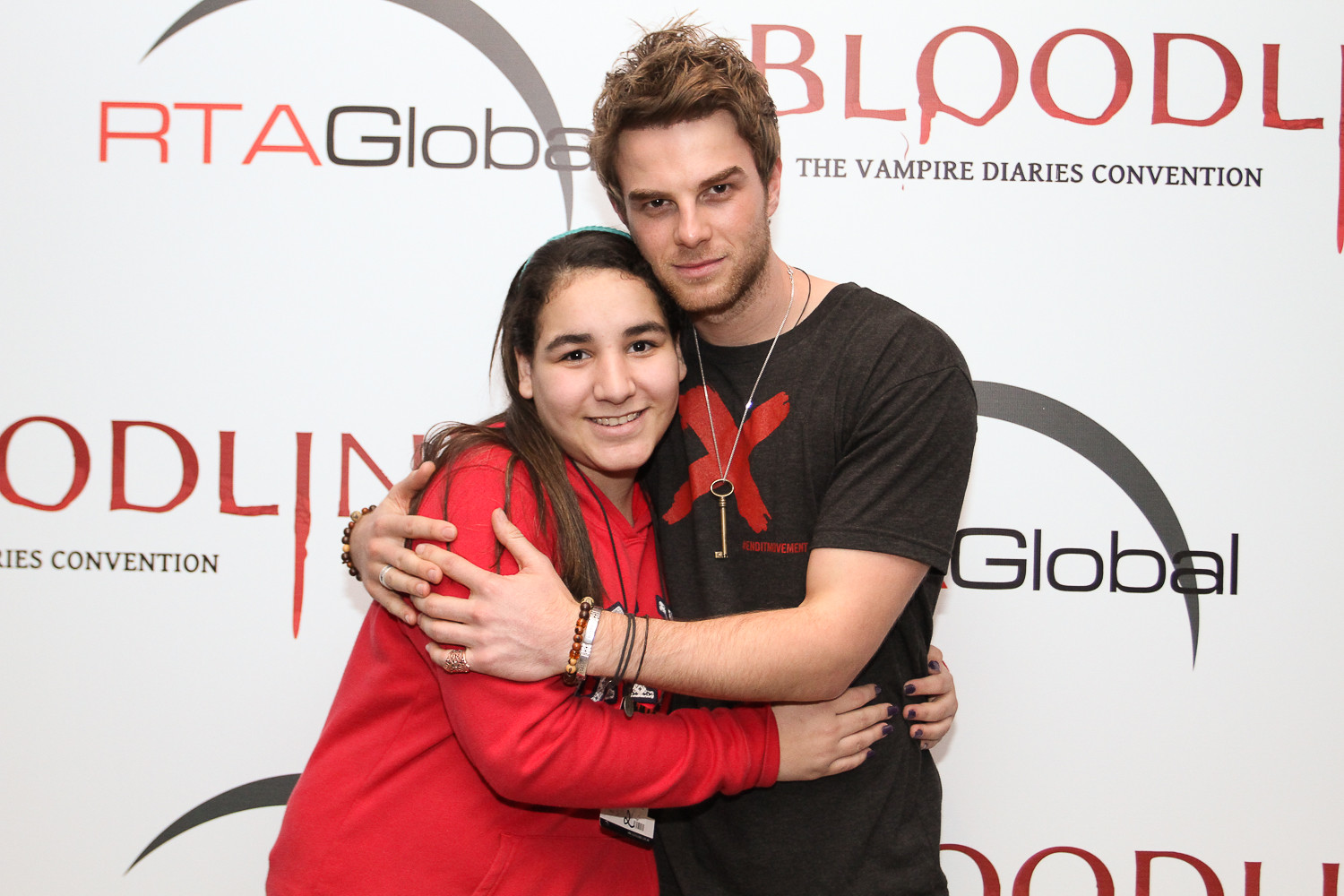In this detailed image, a man and a woman are standing close together, embracing each other warmly. The woman, dressed in a red shirt, is hugging the man's waist while he has his arm around her shoulder. He is wearing a black t-shirt with a prominent X mark on the front and a necklace featuring a gold key. Both are smiling happily for the camera. 

The background consists of a white wall adorned with various promotional logos, specifically for "RTA Global, Bloodline, The Vampire Diaries Convention," indicating that the setting is an indoor event related to the popular TV series. The man, with short hair and a cheerful expression, is looking directly into the camera. The colors in the image include white, orange, gray, red, black, brown, and tan, enhancing the lively and engaging atmosphere of this fan meeting.